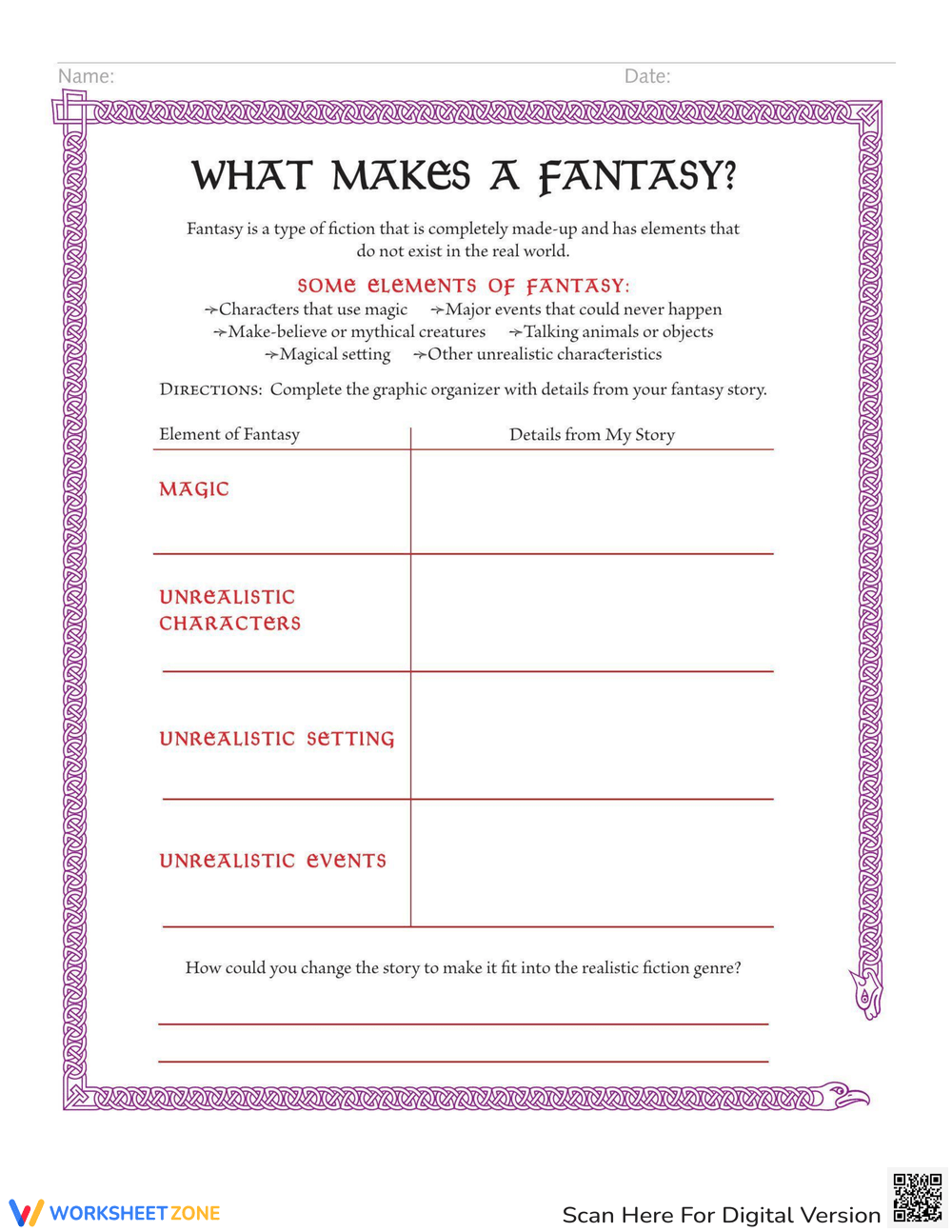The image depicts a vertical rectangular worksheet on white paper, featuring an elaborate Celtic knot border in a purplish hue that frames the entire page, except for the lower right-hand corner where the knot terminates with an intricately rendered eagle head. At the top, the worksheet is labeled in black capital letters: "WHAT MAKES A FANTASY?" Below this heading, in smaller print, is a definition: "Fantasy is a type of fiction that is completely made up and has elements that do not exist in the real world." 

Highlighted in pinkish text, the worksheet lists "Some elements of fantasy:" followed by several bullet points: "characters that use magic, major events that can never happen, make-believe or mythical creatures, talking animals or objects, magical settings, and other unrealistic characteristics." Below these elements, there are directions instructing students to "Complete the graphic organizer with details from your fantasy story."

The graphic organizer consists of a table listing different elements such as "characters," "settings," and "events," with lines provided next to each element for students to add details from their stories. At the very bottom, there's a prompt: "How could you change the story to make it fit into the realistic fiction genre?" followed by space for further student input. In a smaller font beneath this section, the worksheet is branded with "Worksheet Zone" and includes a QR code to access a digital version.